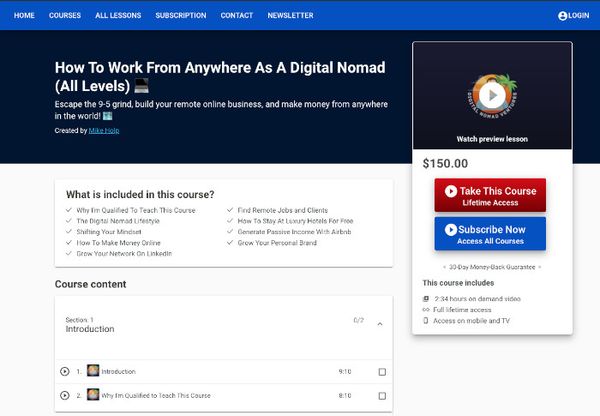At the top of the page, the navigation bar is prominently displayed against a blue background, with white text links on the top left corner including: Home, Courses, All Lessons, Subscription, Contact, and Newsletter. In the upper right corner, the option to Login is available.

Directly beneath, in a darker blue section, white text announces the course title, "How to work from anywhere as a digital nomad," suitable for all levels. An accompanying icon of a laptop adds visual interest. Below this, additional white text promotes the course with the tagline, "Escape the 9 to 5 grind, build your remote online business, and make money from anywhere in the world." The course is noted as being created by Mike Mulp.

In a prominent white box, black text outlines what is included in the course through a two-column bullet list. The headings and items in the list indicate:

- Why I'm qualified to teach this course
- The Digital Nomad Lifestyle
- Shifting Your Mindset
- How to Make Money Online
- Grow Your Network on LinkedIn
- Find Remote Jobs and Clients
- How to Stay at Luxury Hotels for Free
- Generate Passive Income with Airbnb
- Grow Your Personal Brand

Further down, the "Course Content" section is introduced, detailing the course structure starting with "Section 1: Introduction," accompanied by small video thumbnails and a video preview on the right. The course price is listed as $150. Below the price, two call-to-action buttons are displayed: a red "Take This Course Lifetime Access" button, and a blue "Subscribe Now, Access All Courses" button.